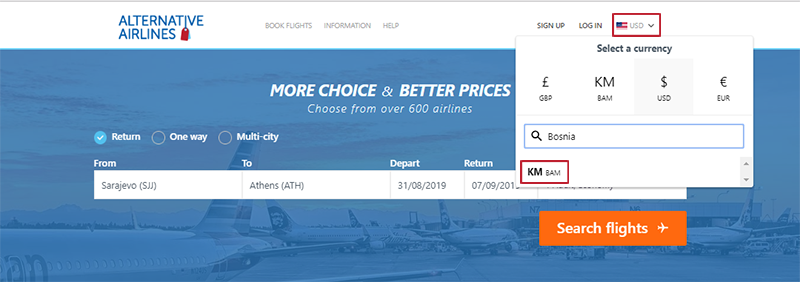This image is a cropped screenshot of an airline booking website. At the top, there's a white banner spanning the width of the page. On the left side of the banner is a logo which reads "Alternative Airlines" in blue capital letters, accompanied by a price tag icon to the right of the word "Airlines." Centered within the banner are three navigation options: "Book Flights," "Information," and "Help," all in small gray text.

On the right side of the banner, there are options labeled "Sign Up," "Log In," and "US Dollars," the latter of which includes a drop-down icon. A red box has been edited over the "US Dollars" option, indicating it has been selected. A drop-down menu has expanded below the "US Dollars" option, displaying a list of currencies with the label "Select a Currency" at the top. The currencies listed include Pound (GBP), Euro (EUR), and Bosnia-Herzegovina Convertible Mark (KM), among others. A search box under the list has the word "Bosnia" typed into it, resulting in the KM currency being highlighted. Another red box is edited over the KM listing, emphasizing the selection process for the Bosnian currency.

The edited red boxes effectively illustrate the user's interaction with the dropdown menu to change the currency setting, specifically selecting the Bosnian Convertible Mark (KM).